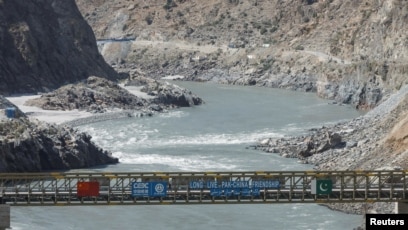This is a color photograph with a dated and washed-out appearance, featuring the watermark "Reuters" in white over a black rectangle in the bottom right corner, indicating it is likely a news agency image. The scene depicts a narrow, straight yellow bridge with side railings, extending over a tumultuous body of light bluish-gray water, which has frothy white waves. The water winds through a rocky canyon landscape with towering, dark and light grayish-brown rocks on either side, though the tops of the rocks are out of frame. The bridge is adorned with several flags: a red flag with a yellow star in the top left corner, a blue flag with white writing, and a long blue flag with the white inscription "Long Live Pan-China Friendship." Additionally, on the right side of the bridge, there is a green flag featuring a white moon and star. This scenery lacks any visible greenery, creating an overall stark and rugged environment. In the background, the surrounding mountain-like rocks further emphasize the harsh and barren nature of the landscape.